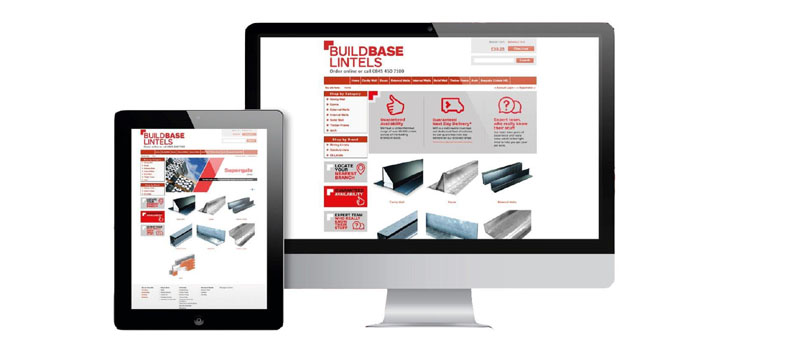In this image, a computer monitor and a tablet are displayed side by side against a plain white background, suggesting the image might be intended for use on a website or as part of an advertisement with no distinct contextual clues. 

On the computer monitor, a retail site is visible, characterized by its white background. In the upper left corner of the screen, the words "BuildBase Lintels" are prominently shown in red block letters. Interestingly, "BuildBase" is merged into a single word, with "BASE" in bold capital letters, while "BUILD" and "LINTELS" are in standard capital letters. Although the other fonts on the screen are too small to be legible, a red background menu bar stretches across the top. Below this menu, there are three distinct gray squares filled with illegible text. 

On the left side of the webpage, a sidebar organizes content into different categories. This sidebar features two red rectangles with white headlines, followed by three smaller rectangles, the top and bottom of which are gray, while the middle one is red.

The tablet screen on the left closely mirrors the layout of the monitor. However, a significant difference is the presence of a large graphic situated just beneath the top menu. This graphic seems to depict two contrasting scenes; one side shows a blue sky with clouds, and the other, though small and unclear, appears to resemble a roof.

This detailed composition provides a glimpse into the structure and design elements of the BuildBase Lintels website, showcasing its primary color scheme and layout consistency across devices.